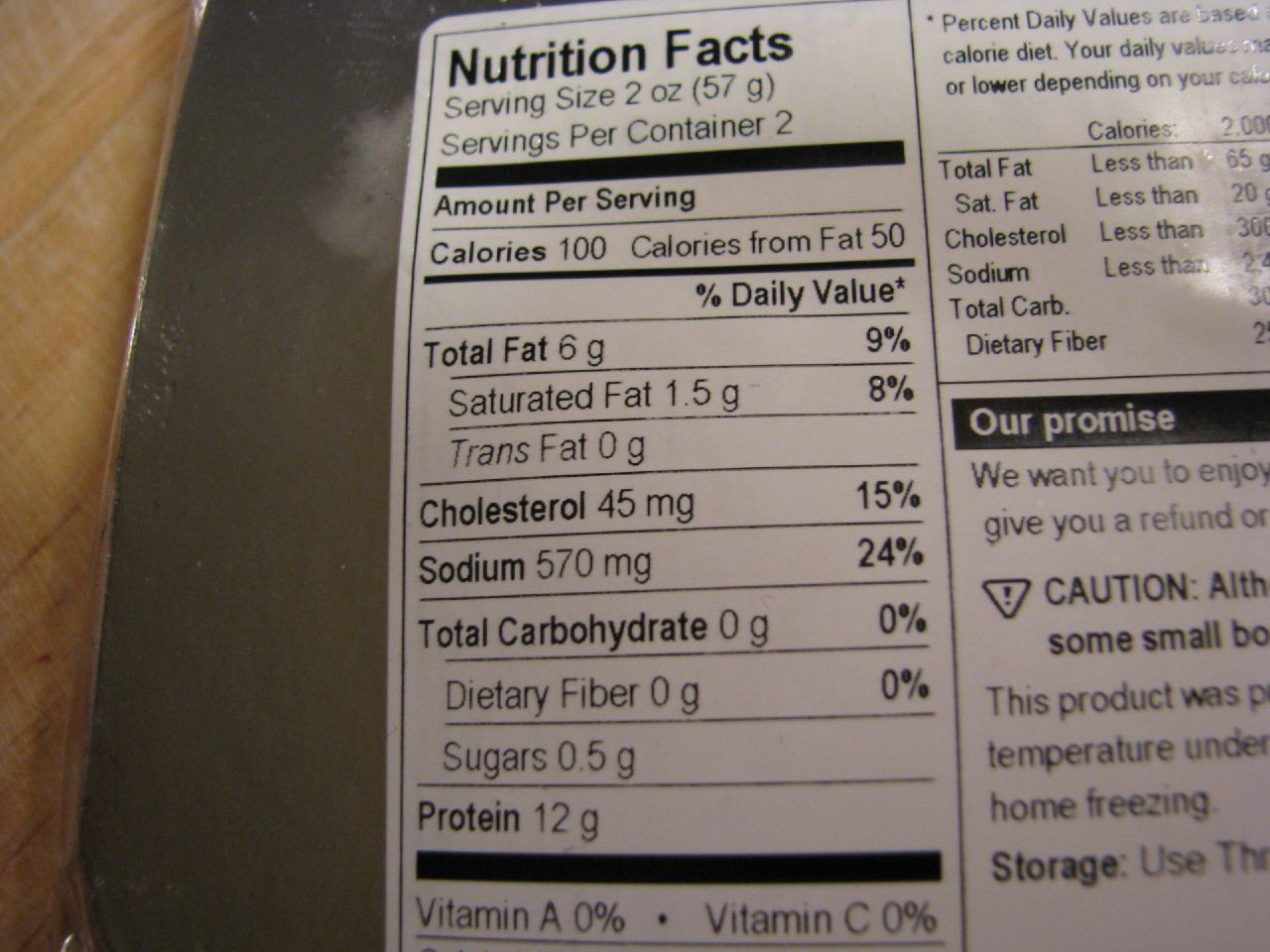This detailed color photograph shows a close-up of a silver food package lying on a wood tabletop, identifiable by the visible wood grain pattern along the left-hand side. The focal point of the image is the white nutrition label with black text, which is partially cut off on the right and bottom edges. The label lists the following details: 

- Serving size: 2 ounces (57 grams)
- Servings per container: 2
- Amount per serving: 100 calories (50 calories from fat)
 
The nutritional breakdown per serving includes:
- Total fat: 6 grams (9% DV)
  - Saturated fat: 1.5 grams (8% DV)
  - Trans fat: 0 grams
- Cholesterol: 45 milligrams (15% DV)
- Sodium: 570 milligrams (24% DV)
- Total carbohydrate: 0 grams
  - Dietary fiber: 0 grams
  - Sugars: 0.5 grams
- Protein: 12 grams

Additionally, it notes vitamins with 0% daily value: Vitamin A and Vitamin C. Just below the nutrition facts, there is text suggesting customer satisfaction and storage instructions, though not fully legible due to the cut-off. The package itself appears sleek against a wooden and possibly a secondary dark laminated surface underneath it.